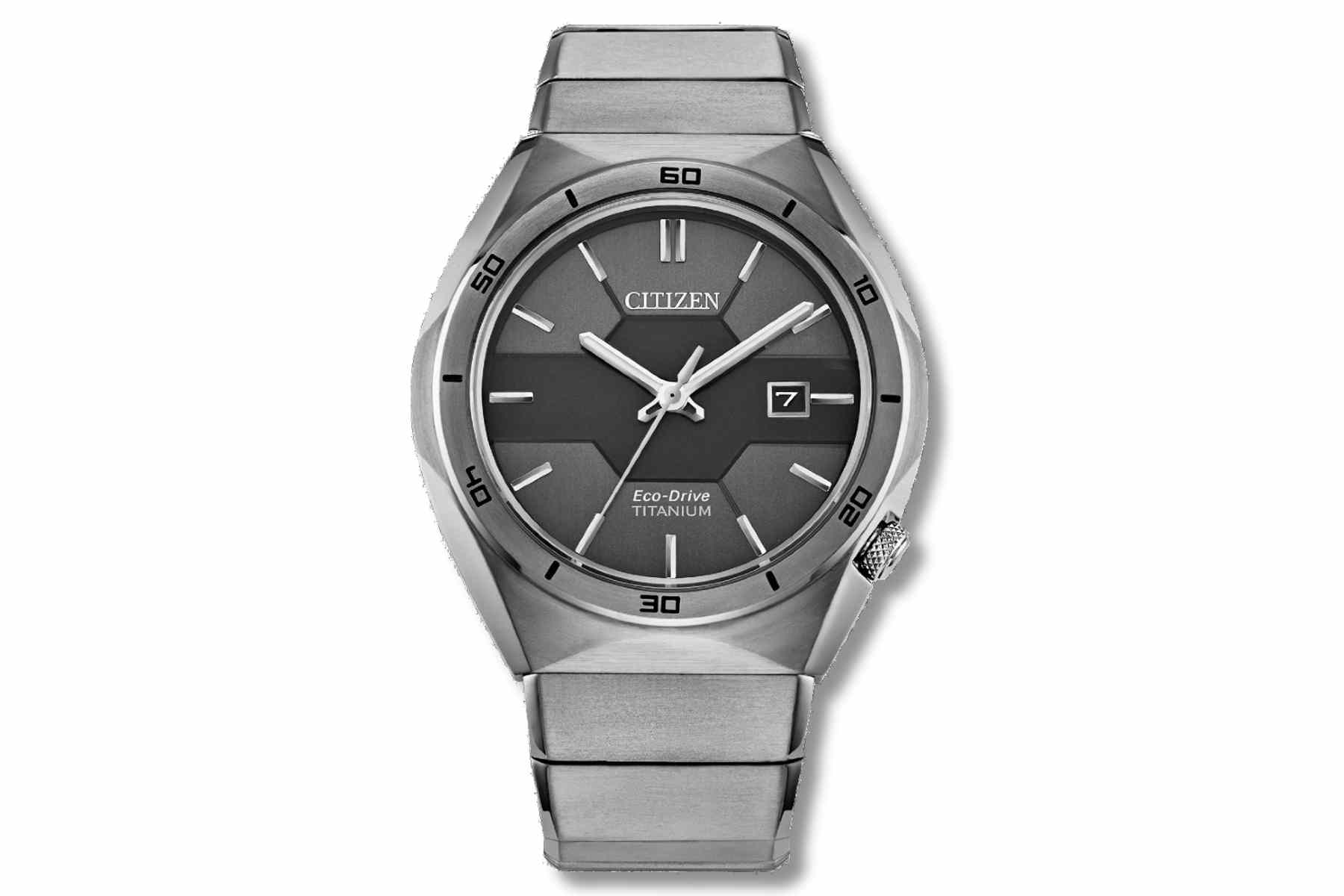A detailed image caption of a man's watch with shared and emphasized details from both descriptions:

The image features a Citizen Eco-Drive Titanium watch prominently displayed against a background. The watch throws a subtle shadow to the right and downward. The watch face is silver, and a metal band partially visible. In place of traditional hour numbers, the watch uses minimalist indicators: two silver slashes for the 12 o'clock position and single slashes for the other hours. Around the outer edge of the dial, specific minute markers are labeled, with '60' above the 12 o'clock, '10' above the 2 o'clock, '20' above the 4 o'clock, '30' at the bottom (6 o'clock), '40' above the 8 o'clock, and '50' above the 10 o'clock positions. The watch's hands include a prominent long hand pointing toward the 10, a shorter hour hand, and a second hand, each contributing to the watch's intricate and precise design.